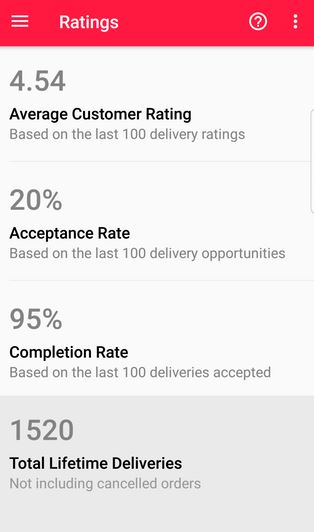This rectangular digital image, designed for a mobile device, presents an interface displaying various ratings and stats likely related to a delivery app. The image is approximately twice as high as it is wide, creating a portrait orientation typical of smartphone screens.

At the top is a cherry red header featuring three short stacked horizontal lines on the far left, which serve as a menu icon. To the right of this icon is the word "Ratings" in white text. Near the top right corner, there is a white circle enclosing a question mark, indicating a help or information button. Further to the right, three vertical dots signal an options menu.

Below the header are four rectangular sections, evenly distributed down the image without clear borders. The top three sections have a very light gray or off-white background. 

1. **First Section**: 
   - **Rating**: "4.54" in a medium gray, bold font at the upper left.
   - **Description**: "Average Customer Rating" in black, bold text immediately below the rating.
   - **Detail**: "Based on the Last 100 Delivery Ratings" in smaller, gray text below the description.

2. **Second Section**: 
   - **Acceptance Rate**: "20%" in medium gray, bold font at the upper left.
   - **Description**: "Acceptance Rate" in black, bold text beneath the rate percentage.
   - **Detail**: "Based on the Last 100 Delivery Opportunities" in smaller, gray text below the description.

3. **Third Section**: 
   - **Completion Rate**: "95%" in medium gray, bold font at the upper left.
   - **Description**: "Completion Rate" in black, bold text below the rate percentage.
   - **Detail**: "Based on the Last 100 Deliveries Accepted" in smaller, gray text below the description.

4. **Fourth Section**: 
   - **Lifetime Deliveries**: "1520" in medium gray, bold font at the upper left. This section has a slightly darker light gray background compared to the others.
   - **Description**: "Total Lifetime Deliveries" in black, bold text beneath the number.
   - **Detail**: "Not Including Cancelled Orders" in smaller, gray text below the description.

This image clearly presents key performance statistics for a delivery service, leveraging a clean and organized layout to ensure easy readability and quick access to important information.